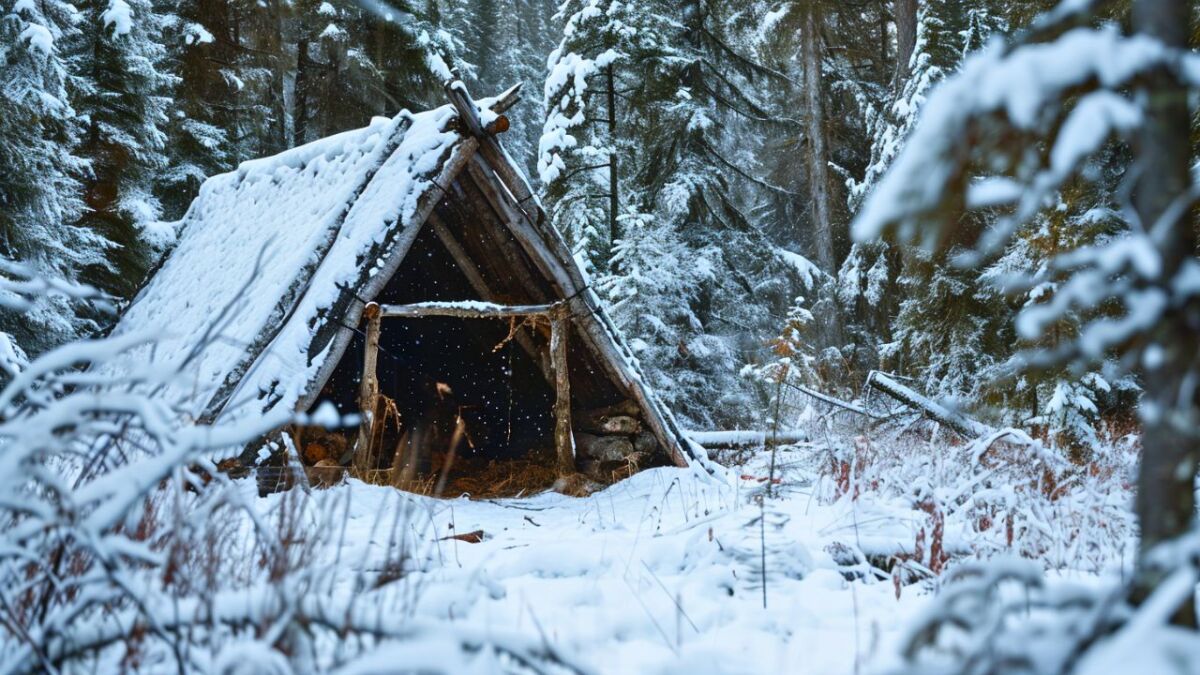The image depicts a serene, wintry forest setting during daylight hours. A thick blanket of snow covers the ground and dusts the branches of numerous evergreen trees in a heavily wooded area. In the foreground, brown grasses poke through the snow, providing a stark contrast to the white landscape. Dominating the left side of the picture is a rustic, handmade wooden structure that closely resembles a triangular lean-to or tent. The structure is formed by logs arranged diagonally to meet at a peak, with an open front that lacks any doors or walls. A hitching post stands in front of this entrance, featuring vertical posts connected by a horizontal beam. The roof of the structure is snow-covered, while the interior remains darker and snow-free. Inside, on the right-hand side, lies a stack of wood, possibly intended for a fire, adding to the impression that this is an outdoor camping shelter.